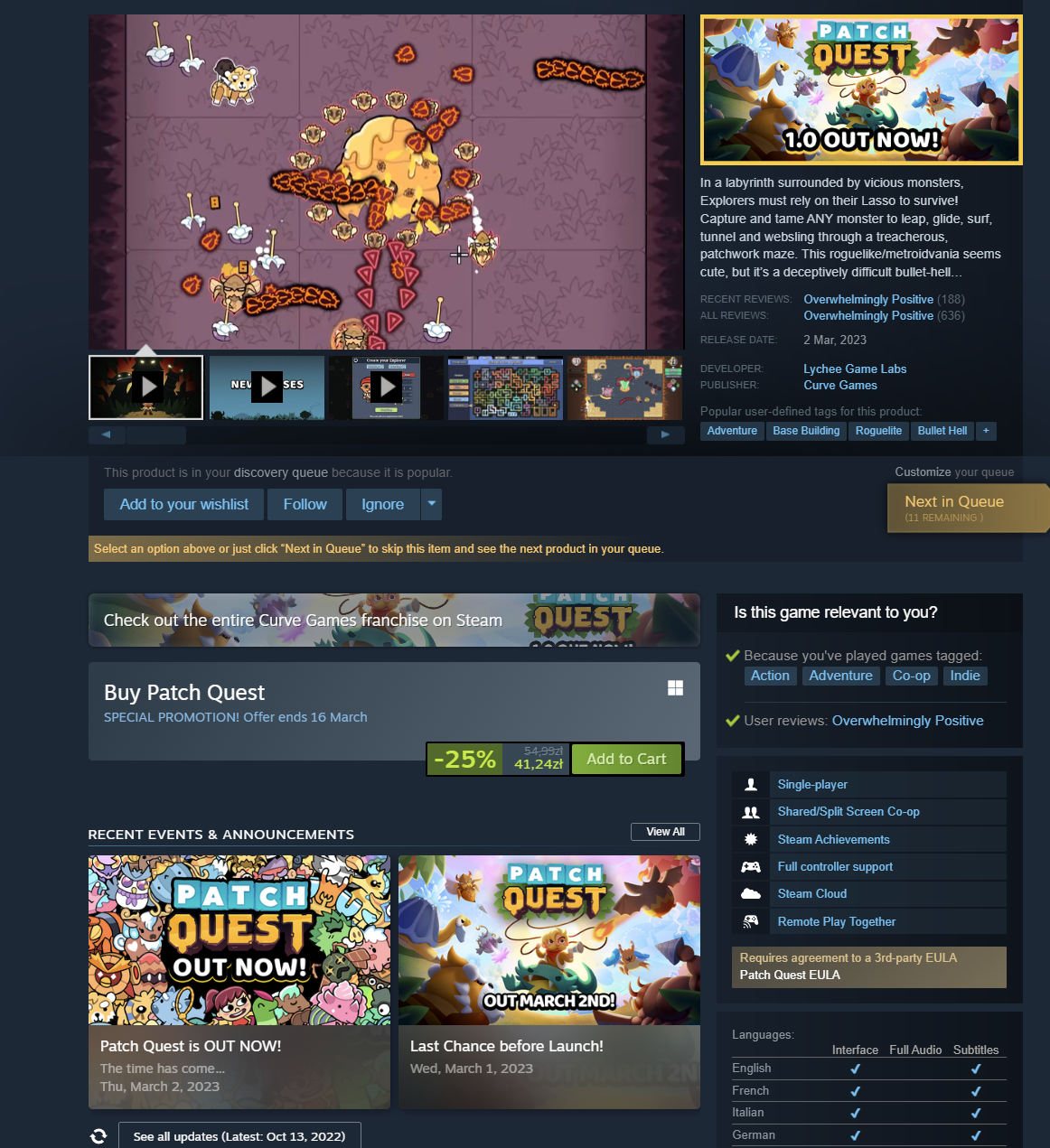The website displays a vibrant advertisement for the computer game "PatchQuest". The page is divided into multiple colorful boxes, each serving a distinct function. In the upper right corner, there's a square featuring the "PatchQuest" logo against a pale blue backdrop adorned with cartoon figures, including what appears to be a fox and a turtle, set against a blue sky with white clouds. Just beneath this logo box is another square containing white lettering, which unfortunately is unreadable. To its left, a larger square with a purple and yellow-orange color theme showcases several avatars from the game, depicting whimsical cartoonish monster figures. Below these main sections, a series of smaller screenshots display black squares with right-facing gray triangles, indicating playable videos for different gameplay previews. Towards the bottom of the page, options to "Add to your wishlist," "Follow," and "Ignore" are presented in an icy blue font, providing interactive choices for the user.